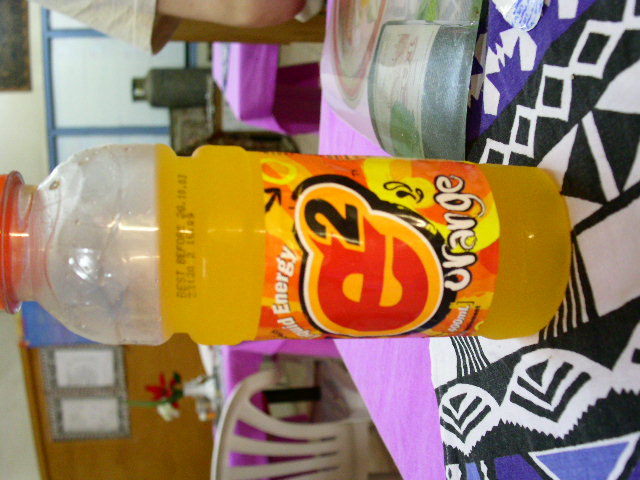A vibrant bottle of orange E2 energy drink, containing 400 ml, is prominently displayed on a tabletop, though the image is rotated 90 degrees to the left. The bottle is made of plastic and contrasts with the purplish-pink tablecloth adorned with tribal-design table runners found in a diner setting. A person's arm, clad in a short-sleeved T-shirt, is partially visible in the frame. In the background, large windows provide natural light, enhancing the indoor ambiance. Several tables are adorned with decorations, including a vase filled with flowers and some salt and pepper shakers.